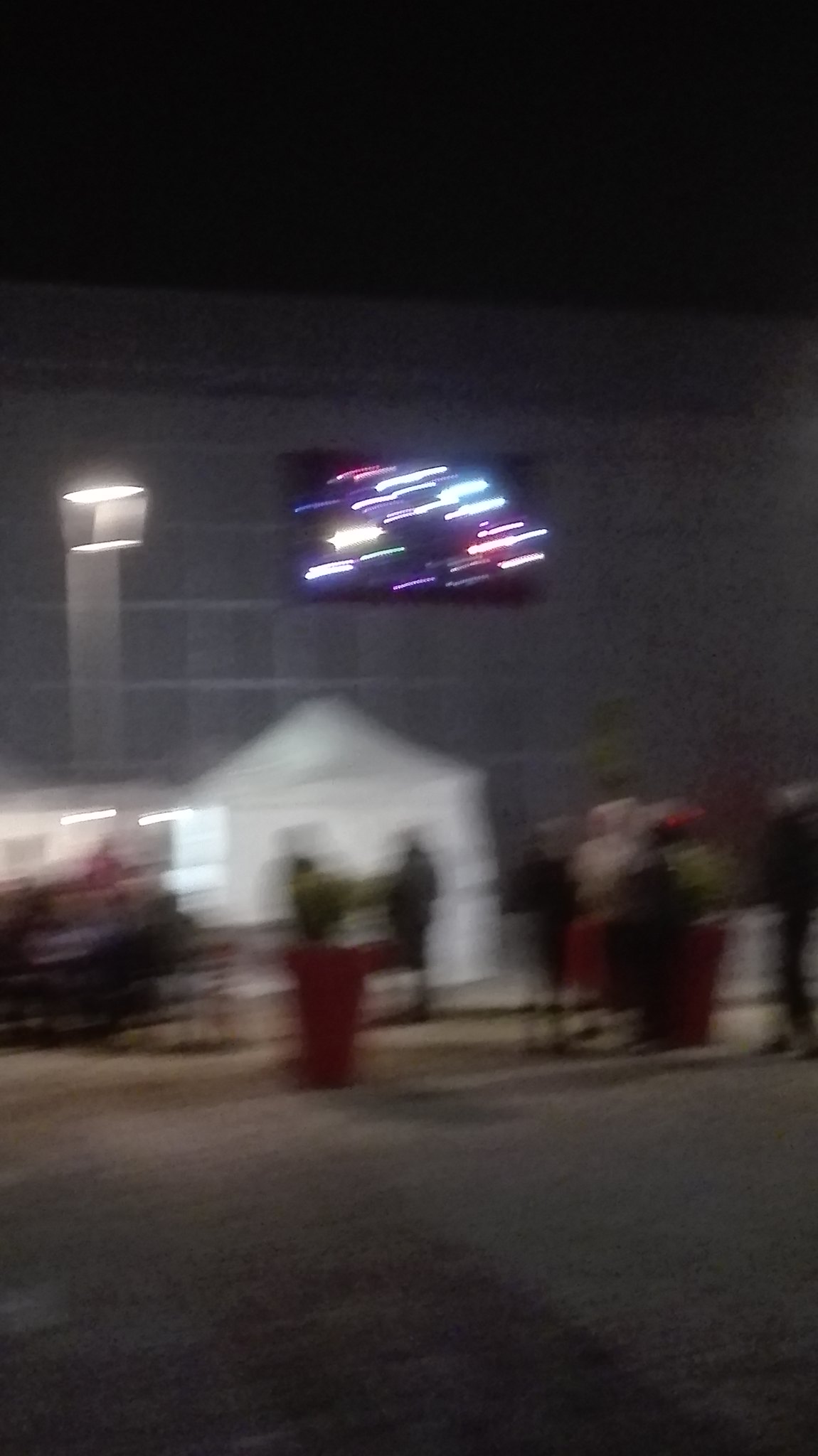A vertical, nighttime photograph captures an outdoor scene with a blurred and streaky effect, likely due to camera movement. The inky black night sky serves as the backdrop, and the setting appears to be a cement-floored patio enclosed by a white cement wall. To the left, a glowing street lamp casts light onto the scene. A large TV or projector screen, mounted on the wall, displays indistinct streaks of bright color. Positioned directly beneath the screen is a white patio tent, accompanied by an arrangement of chairs and tables to its left. In front of the tent, tall red planters filled with bushes add a touch of greenery to the otherwise urban environment.